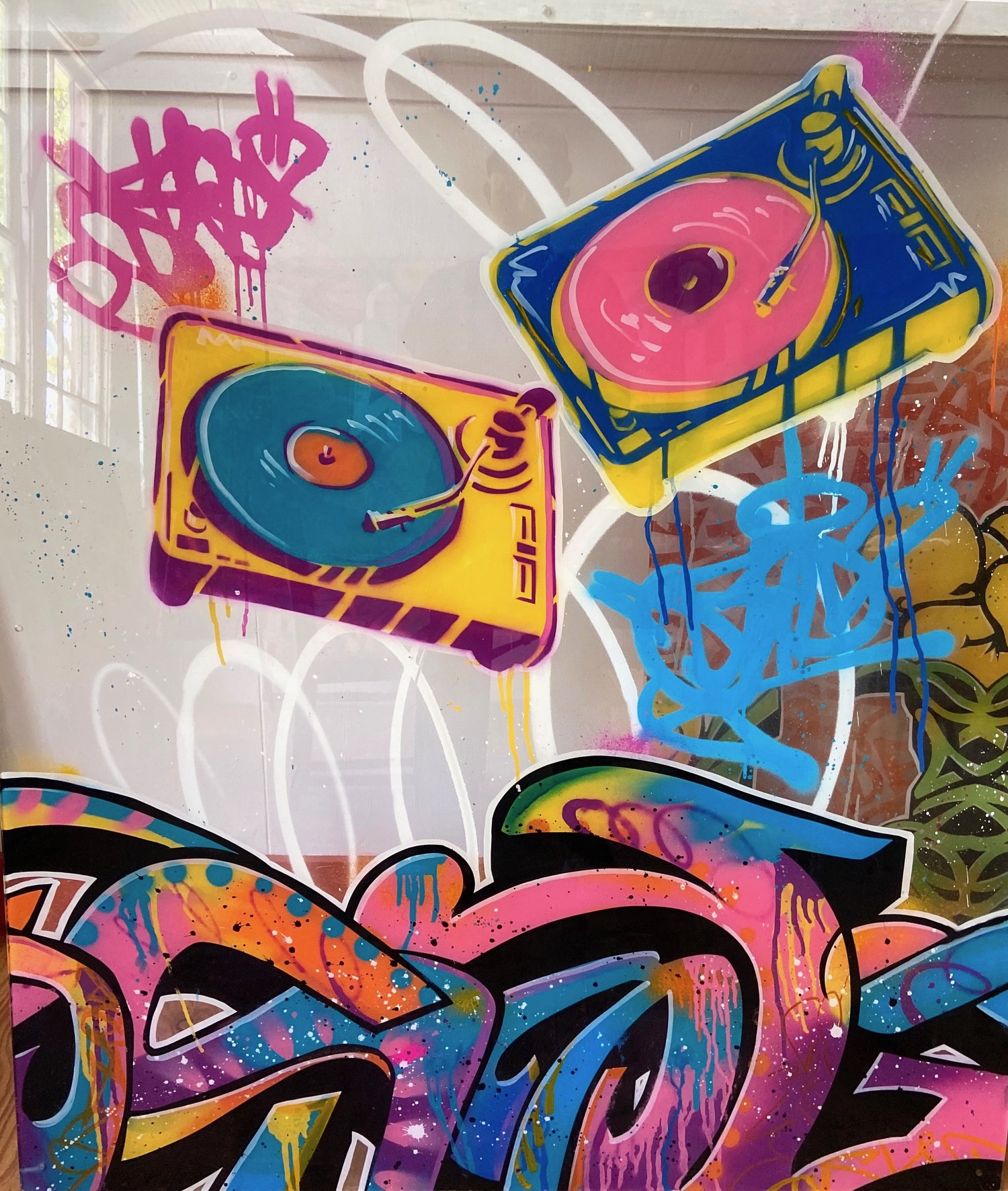This image features a graffiti-covered wall, prominently displaying two distinct record players. The first record player, painted in a blend of purple and yellow, features a blue record with an orange center, and a matching purple and yellow needle arm. The second record player is yellow and blue, holding a pink record with a purple center, with a blue and yellow needle arm. Both record players are positioned diagonally, adding dynamic angles to the artwork. In addition to the record players, the wall boasts a chaotic array of graffiti tags in hues of pink, purple, and orange, with some partially legible letters and shapes. Splashes of white and black outlines accentuate various elements of the graffiti, adding depth to the colorful scene. A drawn window, with light peeking through, is visible in the upper left corner, enhancing the artistic ambiance of the wall. The overall effect is a vibrant and visually engaging graffiti mural, dominated by the detailed renderings of the two record players.